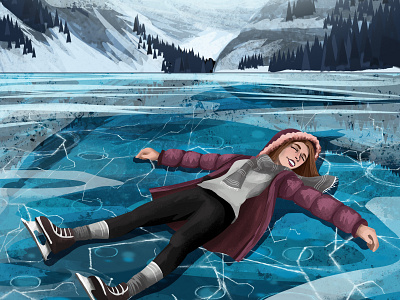This detailed, digital 2D drawing captures a whimsical winter scene of a woman who has fallen while ice skating on a vast, frozen-over lake with visible white cracks. She is lying on her back with her head turned to the right, eyes closed, but smiling, showing she is not distressed. The woman has brown hair and is dressed warmly in black ice skates with silver blades and white laces, gray socks, tight black pants, a white shirt, and a gray scarf. Her vibrant purple parka, adorned with a pink fur-lined hood, stands out against the icy blue foreground. Beyond her, the serene backdrop features snow-covered mountains and black triangle-represented pine trees, creating a picturesque and tranquil winter landscape. The ice on the lake extends far into the distance, shifting from a rich aqua blue near the woman to more whitish hues, where the mountains and trees are reflectively mirrored on the frosty surface.